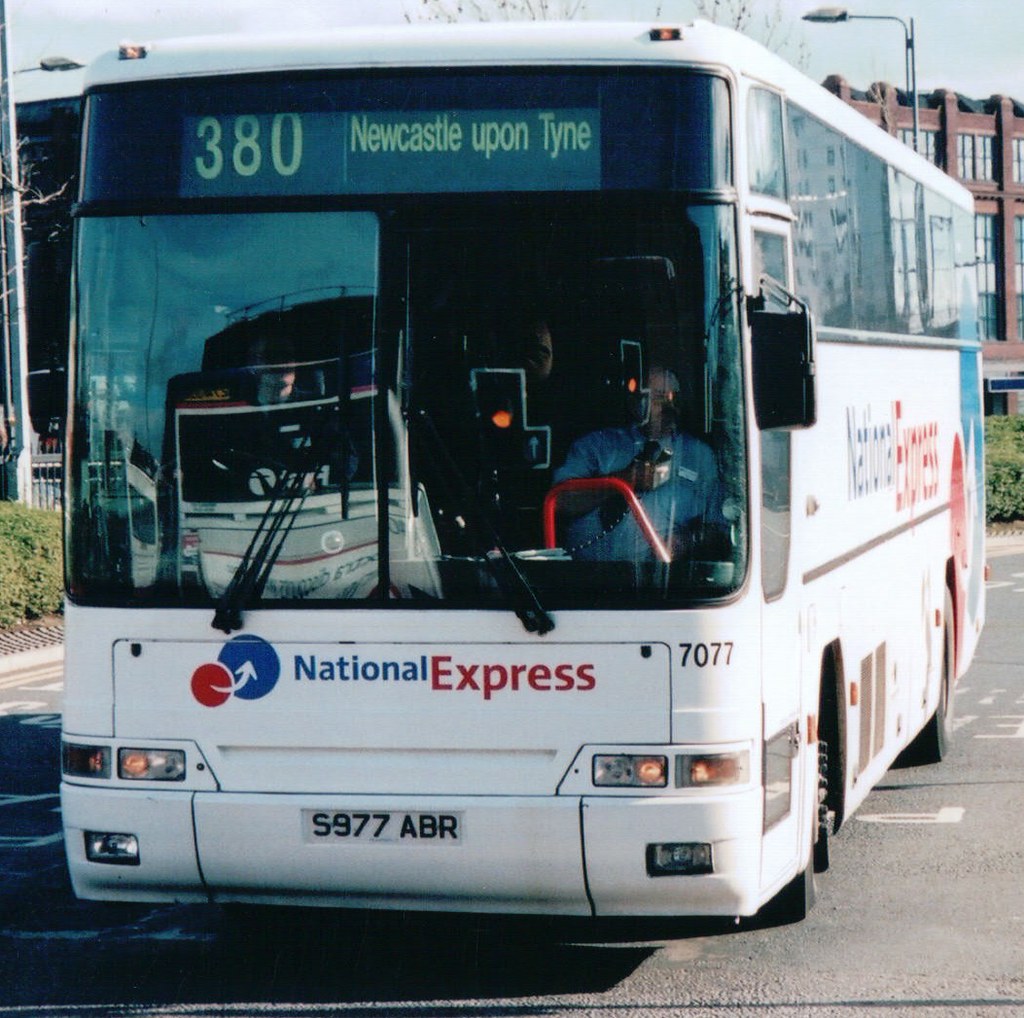The image captures a National Express public transportation bus, akin to a Greyhound bus in the United States, navigating a city street. The white bus prominently displays the company’s logo, characterized by interlocking red and blue circles. The destination "380 Newcastle-upon-Tyne" is clearly marked at the top of the bus, which also bears the European license plate S977ABR. A red brick factory-like building serves as the backdrop, with minimal vegetation visible on either side. The male, Caucasian bus driver can be seen talking on a CB radio, likely communicating with passengers. Overall, the photo gives off a slightly vintage vibe, possibly from the 1980s, as suggested by the resolution and color tones.